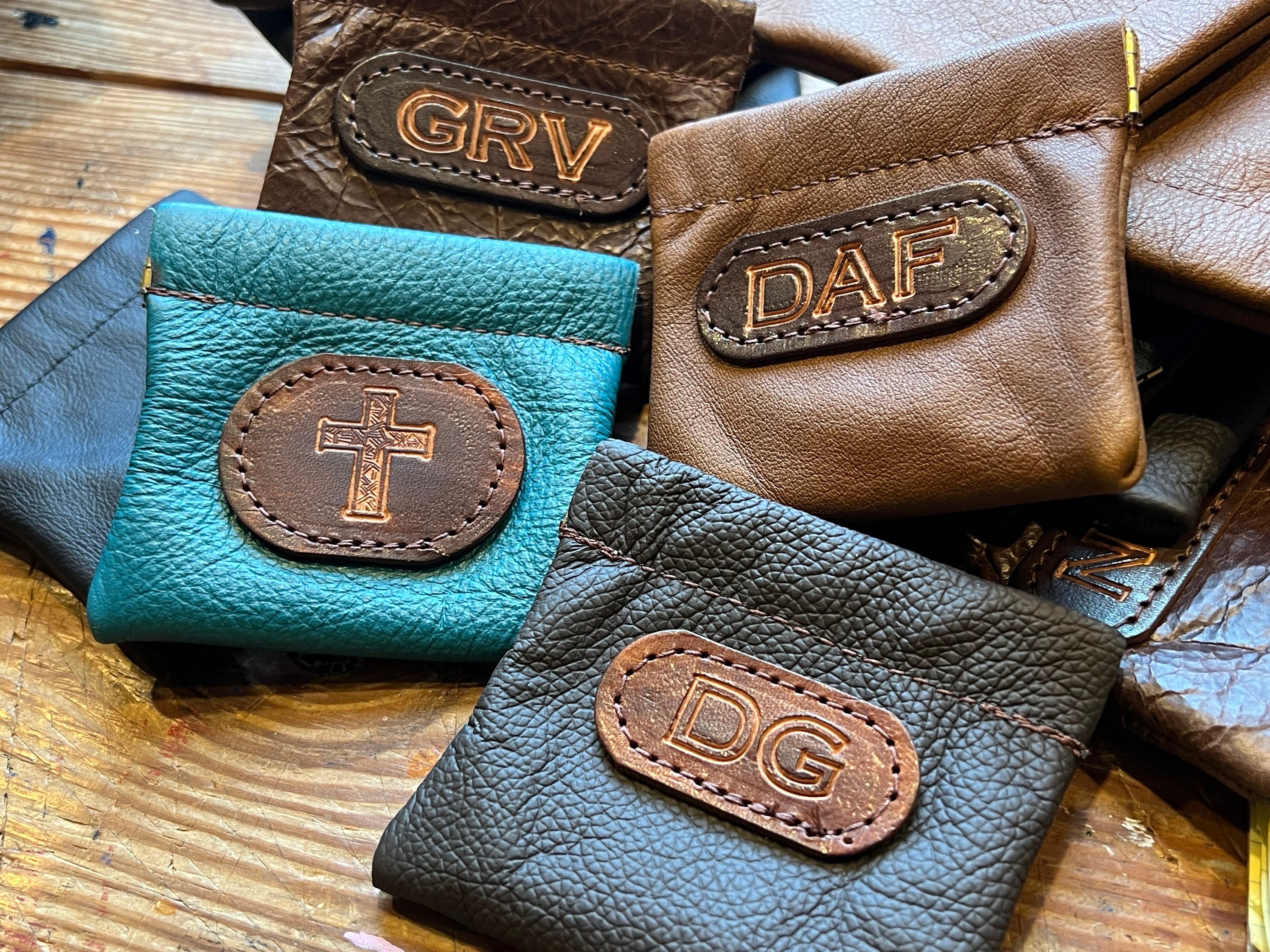The image depicts a collection of leather purses or small bags, numbering around six or seven, neatly arranged on a brown wooden platform. On the left side, there's a dark blue purse. Above it is a light blue purse adorned with a brown design featuring a prominent Christian cross. Further up, a brown bag displays the letters "GRV" in capitalized form. Next to it, another brown bag is marked with the letters "DAF." Below, there is a dark blue purse with the letters "DG" inscribed on a brown strip. Another purse with the letter "N" can also be seen towards the side. Each item bears distinct logos or inscriptions, highlighting a variety of styles and designs. The wooden platform serves as a contrasting backdrop, enhancing the display of these elegantly crafted leather accessories.